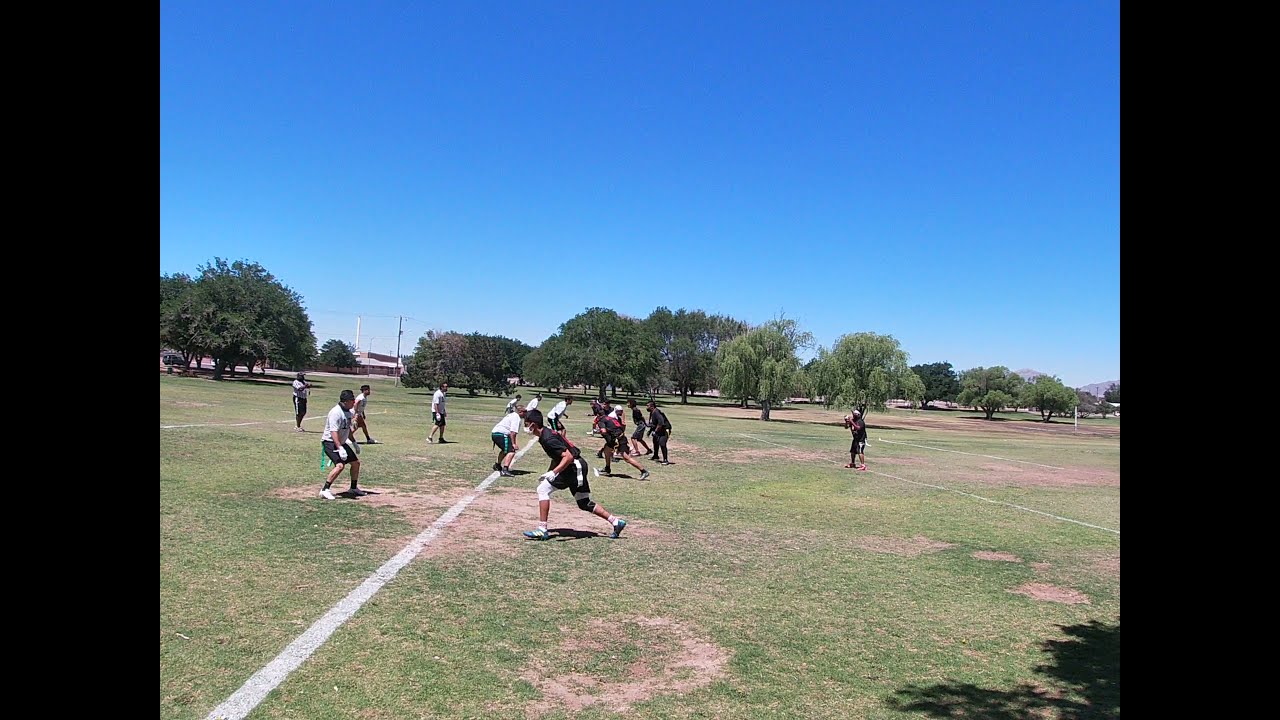In this outdoor image, a group of men, possibly adults and teenagers, appear to be playing a sport that could be soccer or another field game, though no goals are visible. The scene is set in a wide-open park with multiple white lines painted on the grass, including a prominent one running from the lower left toward the middle of the image. The players are divided into two groups on either side of this central line, with one individual standing directly on it, suggesting he may be the referee. The participants are leaning forward or running toward each other, and one person on the left side is holding a ball. They are wearing various protective gear such as knee pads, gloves, and in one case, a hygiene mask. The ground features both grassy areas and dry patches of dirt. The players are dressed in different colored outfits, including black and white with dark shorts. The image is framed by a background of lush green trees, and the upper half is dominated by a clear blue sky with no clouds in sight. A partial tree shadow is visible in the bottom right corner.